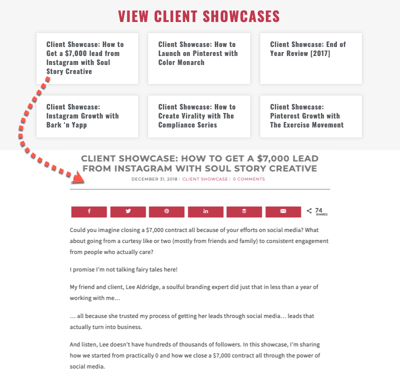Here is a refined and detailed caption based on the provided description:

---

**Detailed Breakdown of Digital Marketing Case Studies**

The image is a screenshot displaying various client showcases, prominently titled at the top in red with the text "View Client Showcases." The showcases offer step-by-step insights into successful digital marketing strategies. Key headings include:

1. **How to Get a $7,000 Lead from Instagram with Real Sole Story Creative**: Highlighting strategies for leveraging Instagram to secure substantial leads.
2. **Client Showcase: Pinterest Marketing with Color Monarch**: Insights into maximizing reach and engagement on Pinterest.
3. **End of Year Review 2017**: A comprehensive look back at the marketing efforts and achievements throughout the year.
4. **Instagram Growth with Bark and Yap**: Techniques for organically growing an Instagram following.
5. **Creating Virality with The Compliance Series**: Steps to generate viral content.
6. **Pinterest Growth with Exercise**: Methods for achieving consistent growth on Pinterest related to fitness.

An arrow pinpoints the first showcase about obtaining a significant lead from Instagram, delving deeper into the methods used. The scenario imagines successfully closing a $7,000 contract through social media engagement, emphasizing the importance of maintaining consistent and meaningful interactions, primarily sourced from friends, family, and dedicated followers.